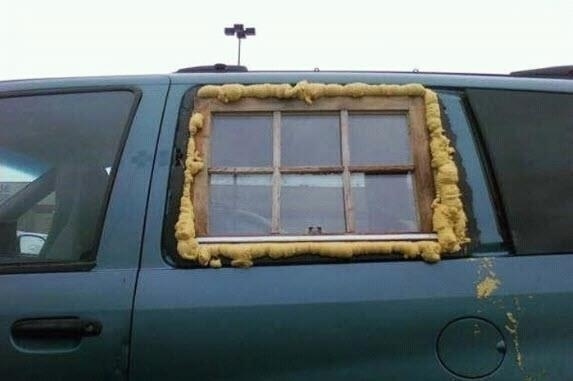The image captures a close-up of the side of an old, blue vehicle, possibly a van, set outdoors under a white sky. The setting appears to be a parking lot, as implied by the full view of the sky and lack of surrounding structures. Notably, the passenger-side window is broken and has been makeshift replaced with a wooden frame, resembling a window from a barn or shed. This DIY repair job is accentuated by a conspicuous yellow substance, likely spray insulation or glue, smeared and leaking around the edges of the window, dripping down onto the vehicle and even onto the gas cap. The foreground includes the car door handle and the gas tank, while above the car, there's a street lamp featuring four downward-pointing square lights. The predominant colors in the image are blue, white, black, yellow, green, tan, and gold, contributing to an overall humorous and makeshift aesthetic.